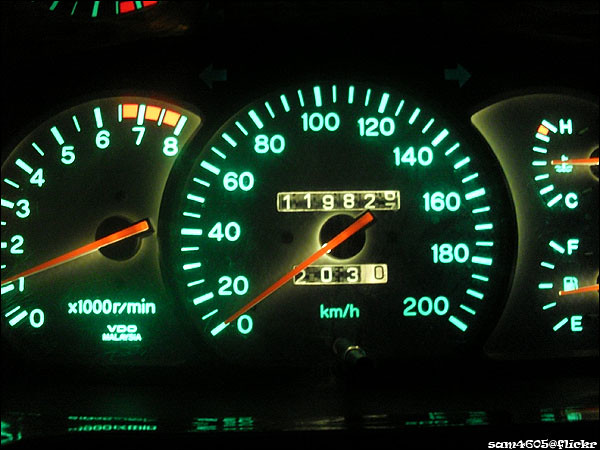A dimly lit image captures the analog dashboard of a stationary vehicle during nighttime. The dashboard is illuminated with a green luminescent glow, highlighting various gauges, including the RPM, speedometer, oil temperature, and fuel level. The speedometer and RPM gauge hands are accented in red, indicating the vehicle is in park with an idle RPM of 1,000 and a speed of 0 km/h. The fuel gauge shows a half tank of gas, and the oil temperature is within the normal range. The odometer reads 119,827 kilometers, with a trip distance of 203 kilometers logged. The scene suggests a potentially older model car, likely situated in Europe or Canada, given the metric measurements.